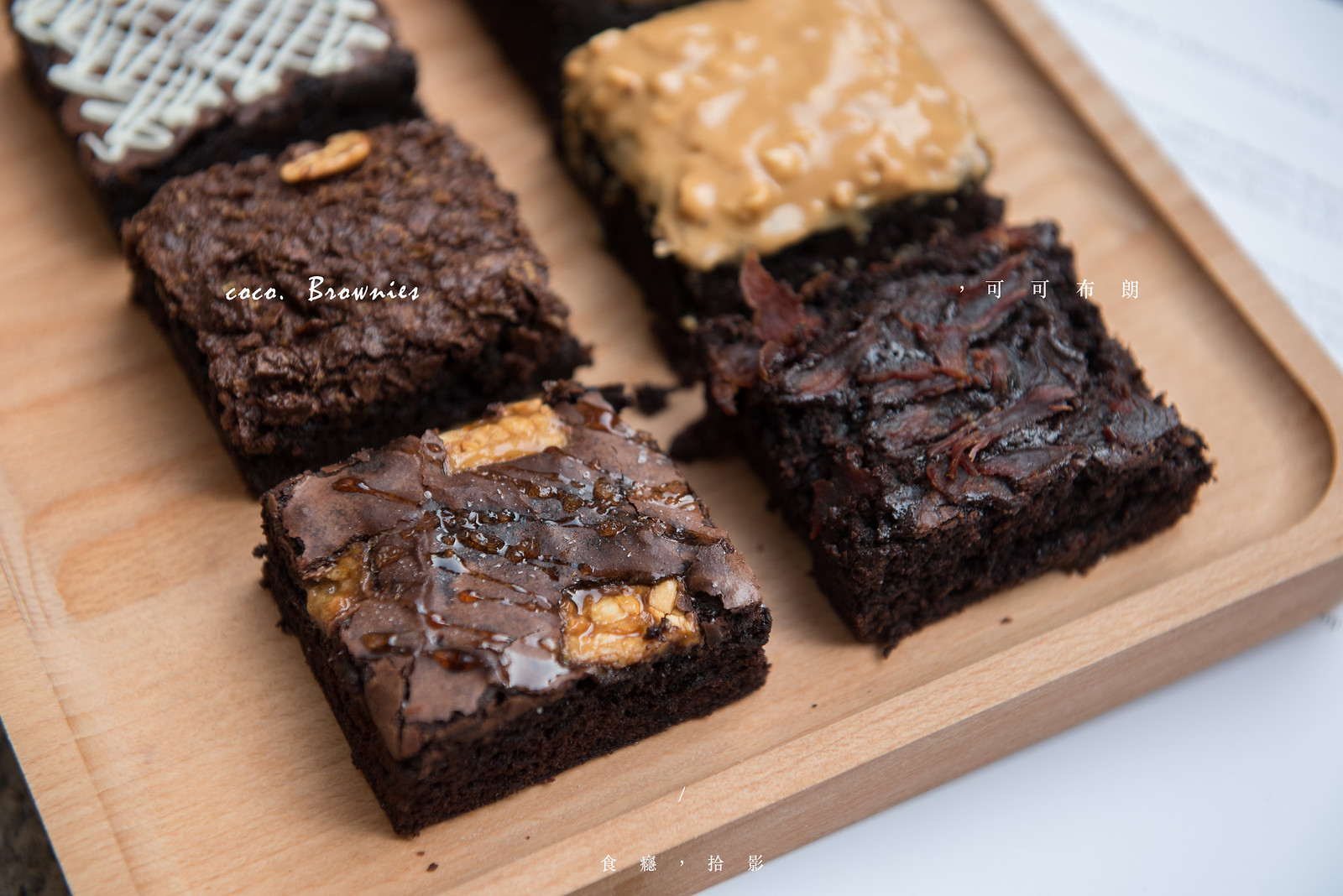A tray of assorted brownies is artfully presented on a rectangular wooden board with a rounded indentation at the center, perfectly crafted for food photography, possibly for a website or blog. The tray rests on a sleek marble countertop, primarily white with a hint of gray in the upper right corner. Overlaying the image, white text on the left reads "cocoa. brownies." alongside some intricate Chinese characters. There are six visible brownies, each with unique toppings and styles. Starting from the upper left, the first brownie features a dark brown base with a delicate crisscross pattern of white icing. Below it, the middle left brownie is mostly brown with a grainy texture and a lone cashew-shaped light brown spot. The lower left brownie is predominantly dark brown, interspersed with light brown patches. The middle right brownie is notable for a light brown paste, reminiscent of peanut butter, covering its surface. Adjacent is the lower right brownie, which sports a mysterious reddish-brown topping. Lastly, peeking slightly from the upper right, a small corner of another brownie is visible, hinting at more delectable varieties.